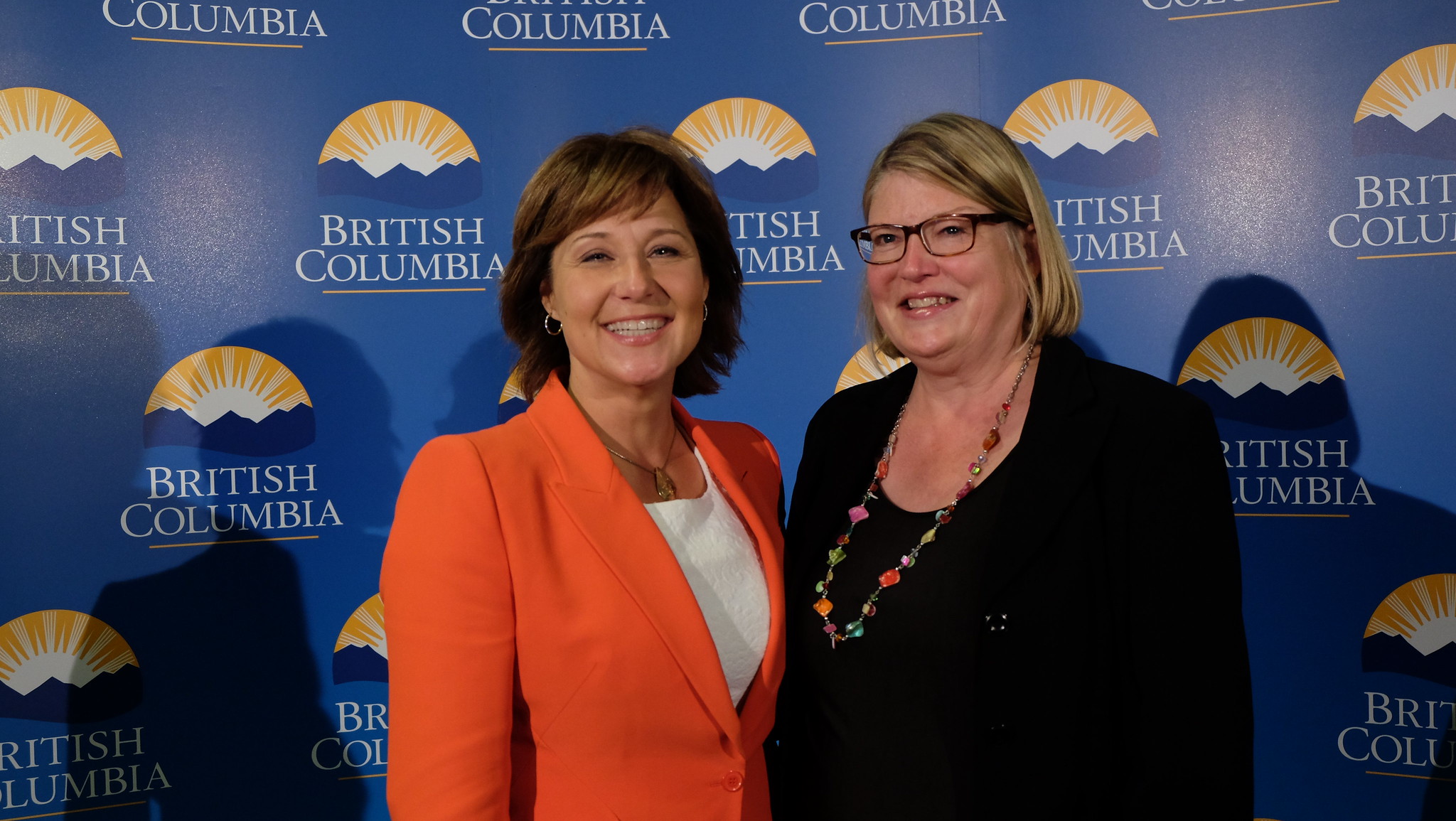The image features two women standing side by side against a blue background decorated with multiple duplications of the British Columbia logo, which comprises yellow sun rays atop navy blue mountains and the words "BRITISH COLUMBIA" in white capital letters.

The woman on the left, appearing to be in her 40s or 50s, has dark skin and short, neck-length dark brown hair. She is dressed in a bright orange blazer over a white blouse. Her accessories include a silver teardrop-shaped necklace, two small hoop earrings, and a pair of hoop earrings.

The woman on the right is slightly larger and also appears to be in her 40s or 50s. She has blonde hair and wears brown glasses. Her outfit consists of a black top, possibly paired with a black cardigan or blazer. She accessorizes with a long, multi-colored necklace featuring beads in shades of purple, green, yellow, and blue.

Both women are smiling and posing pleasantly for the photograph.